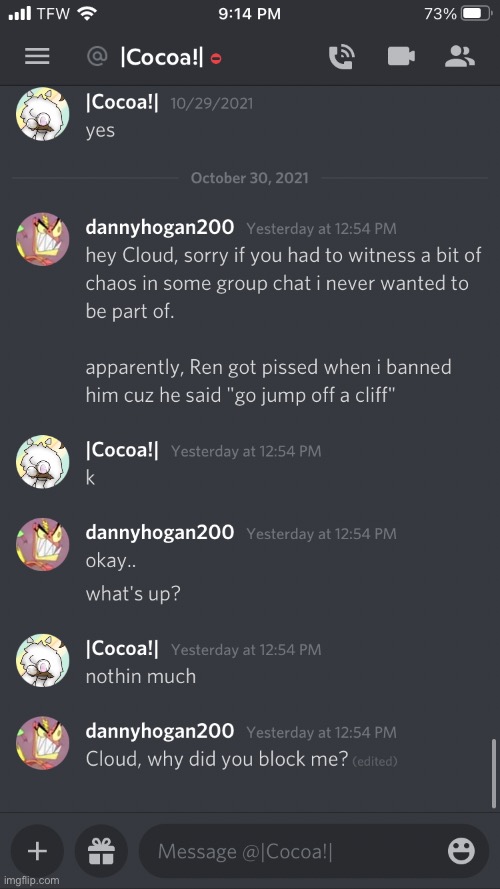Screenshot of a messaging interface with a gray background, timestamped at 9:14 PM, showing a battery level at 73%. The interface features a hamburger menu icon and a top bar with “cocoa!” accompanied by an exclamation mark and an X symbol. There’s also a phone camera icon and an outline of two people representing a profile icon.

The screenshot captures a conversation thread. The first message is from a user named Danny Hogan, with a profile picture resembling an animal, dated October 29, 2021. His message, posted "Yesterday at 12:54 PM," reads: "Hey Cloud, sorry if you had to witness a bit of chaos in some group chat I never wanted to be part of. Apparently, Rin got pissed when I banned him because he said, in quotation marks, 'Go jump off a cliff.'"

Following this, there are replies between Danny Hogan and another user named Coco K, marked by alternating profile pictures. Danny Hogan’s profile picture resembles a monster. Coco K’s first reply, also timestamped "Yesterday at 12:54 PM," says: "Okay, okay, ay what's up." Danny Hogan responds quickly at the same timestamp, "Nothing much. Nothing."